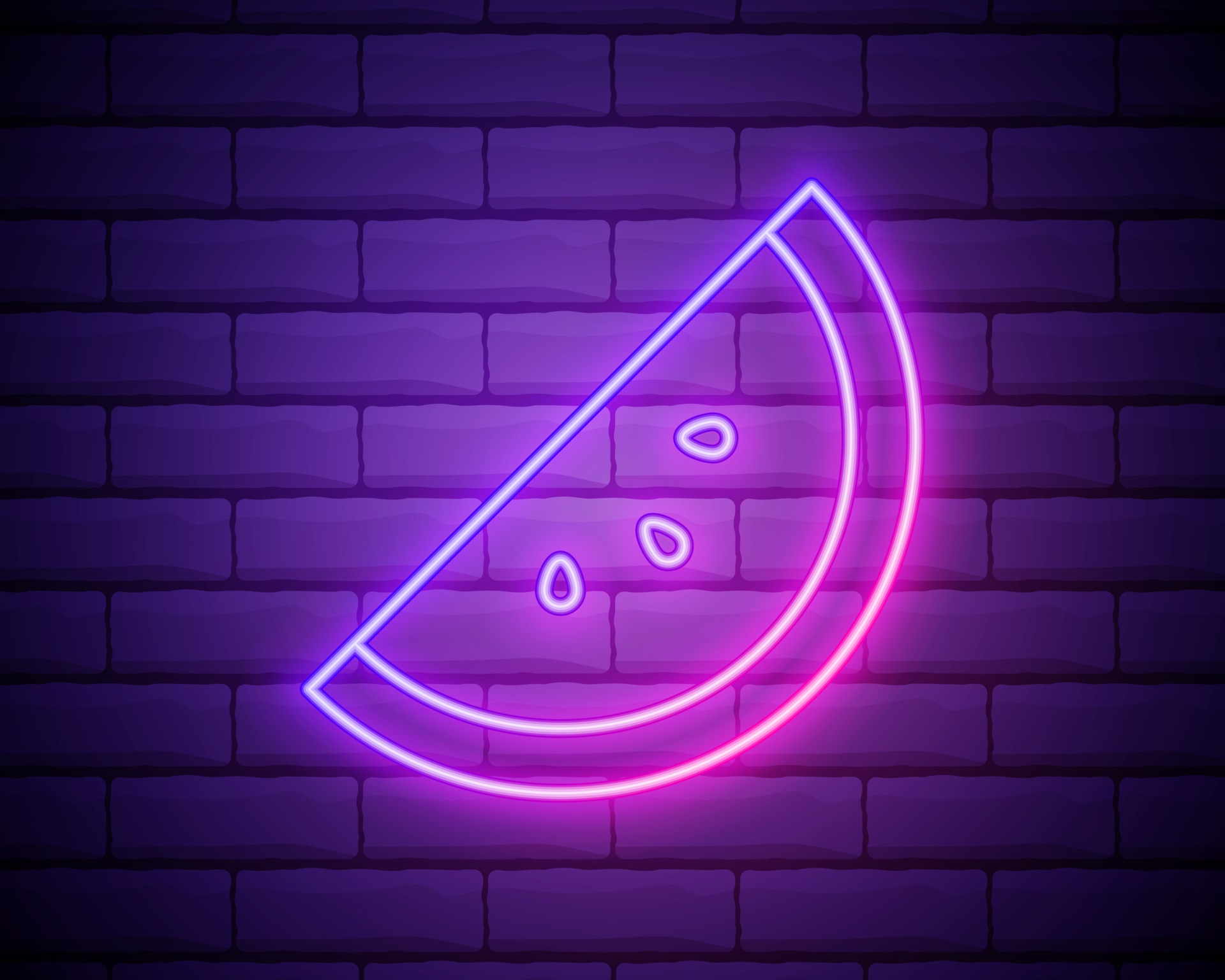This indoor computer-generated image showcases a vividly illuminated neon sign depicting a simplistic, stylized slice of watermelon. The neon sign exhibits a semicircular design featuring a diagonal orientation, with a blue rind that transitions smoothly into a pinkish center. Within the semicircle, three oval shapes represent watermelon seeds glowing in a mix of white and light purple hues. The sign stands out brilliantly against a purple brick wall backdrop, which appears slightly fuzzy around the edges, contributing to an AI-generated aesthetic. The bricks display a gradient from light purple to dark purple, with the very top and bottom edges fading into black. The overall scene lacks textual elements, emphasizing the striking contrast between the fluorescent neon colors and the softly gradated brick background.